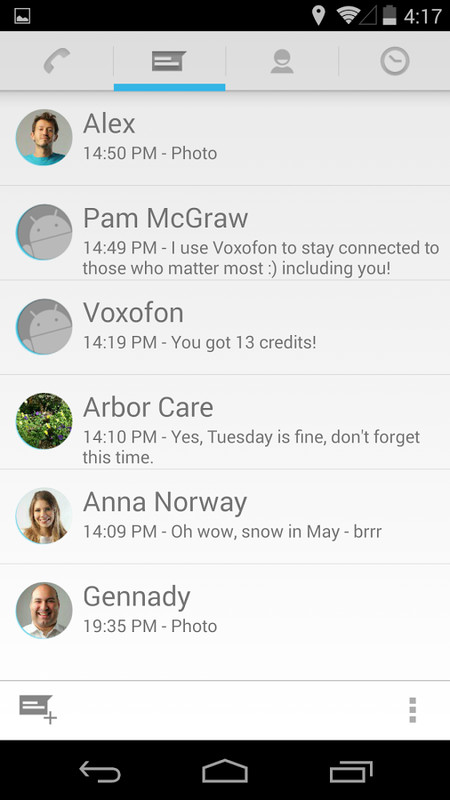The image depicts a screenshot with several distinct sections and graphical elements. At the top of the screenshot, there is a black banner, beneath which is a small square icon in light gray featuring an illustration resembling mountains or hills. Adjacent to this icon are symbols indicating location, Wi-Fi signal, cellular signal, battery status, and the current time displayed as 4:17.

Most of the screenshot's background is a light gray color. The first banner at the top includes icons for phone, messenger, a clock, and a person depicted as an outline drawing. Below this top banner, the screen is segmented into six user profiles. The first profile belongs to Alex, accompanied by his photo. The second profile is for Pam McGraw, represented by a robot icon within a gray circle. Next is a user named Voxophon, spelled in all caps as V-O-X-O-F-O-N. Following Voxophon is Arborcare, spelled A-R-B-O-R-C-A-R-E, and then Anna Norwy. The last listed user is Gennady, spelled G-E-N-N-A-D-Y.

At the bottom of the screenshot, there is another black banner featuring several icons: an arrow pointing left, a house, and two stacked rectangles. The overall impression is one of a contact list or a messaging application interface, organized with informational and visual clarity.